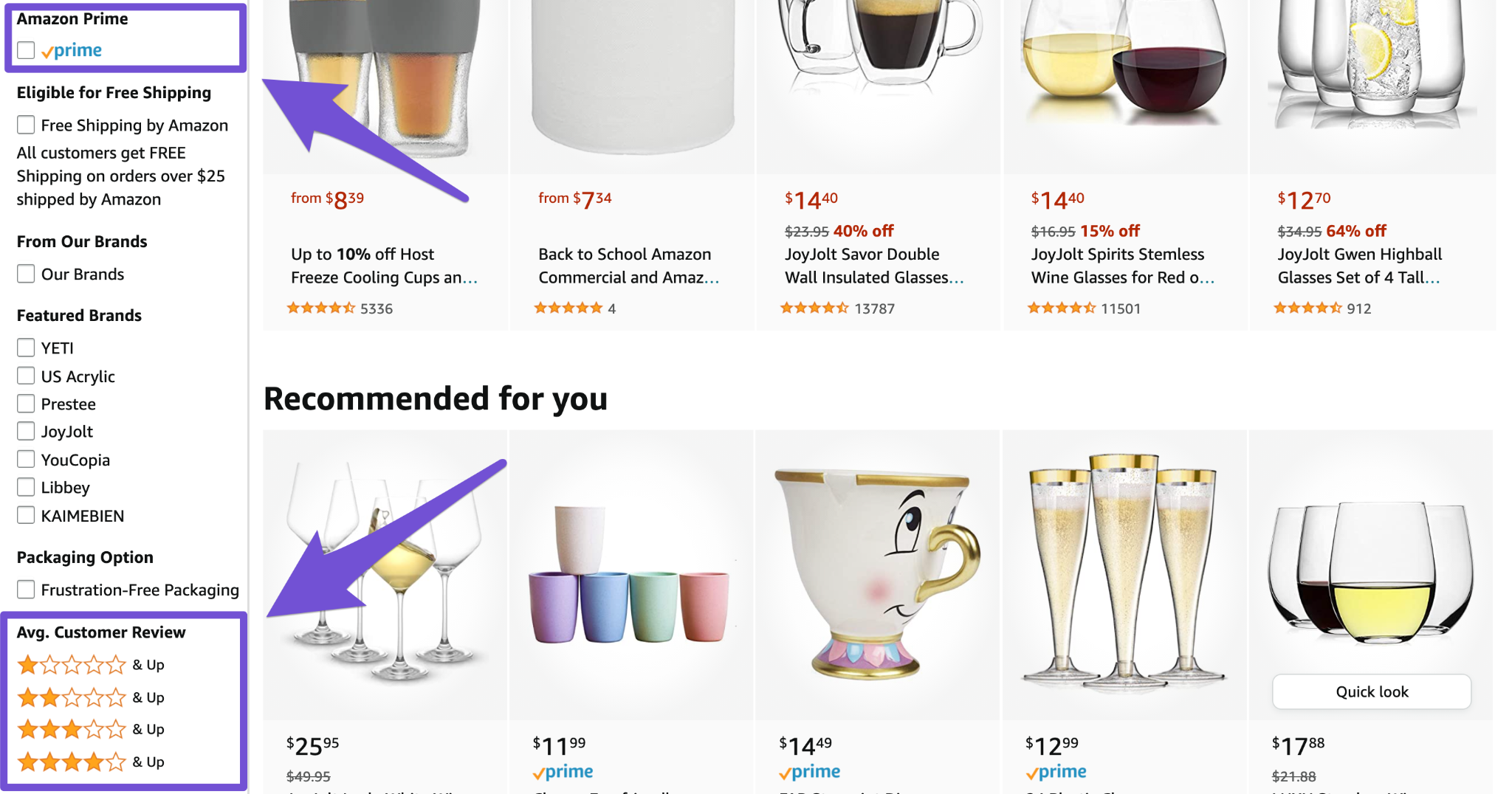"Capturing the essence of premium glassware options available on Amazon, this descriptive image highlights a diverse selection for customers. Featured brands include Yeti, U.S. Acrylic, Prestige, Royal Jewel, Eucopia, Libby, and Cameroon. Showcasing various packaging illustrations with a prominent blue square in the background, representing the average customer view, the image boasts detailed ratings with half gold stars indicating superior quality.

Pricing ranges from $7.34 for back-to-school promotions to $17.88 for high-end wine glasses. Special offerings include up to 40% off on Jolly Jolts, with items like double wands lighting glasses and spray stimulus wine glasses starting at $14.40. Additionally, George Lockwood highball glasses are available at $4, alongside teacups adorned with golden handles and flowery petals for $14.49.

This comprehensive overview emphasizes the value and variety of products eligible for free shipping on Amazon Prime, ensuring all customers get the best deals on orders over $24. Prime benefits include reduced costs, extending from $8.39 up to 10% off on post-freeze cooling cups, ensuring both affordability and elegance for discerning shoppers."